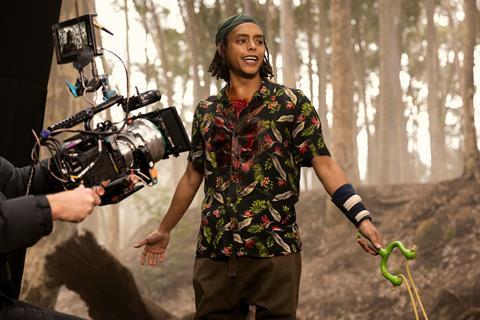The photograph features a black man with chin-length dreadlocks and a green headband, standing in the center of a wooded area, likely a gully with tall trees in the background, on a bright but cloudy day. He is attentively looking to the right and appears engaged in action, possibly from a TV show. He is dressed in a vibrant, multicolored Hawaiian shirt with a black base and green and gray patterns, paired with brown slacks. His left wrist sports a noticeable black wristband with two white stripes. In his left hand, he holds a green slingshot with a yellow sling, poised as if he had just used it. The man has some blood on his neck and shirt, adding an element of intensity to the scene. To his left, partially cropped from the image, another person, likely Caucasian, is seen handling a large, complicated camera rig complete with various cords and a boom microphone, capturing the man's actions.